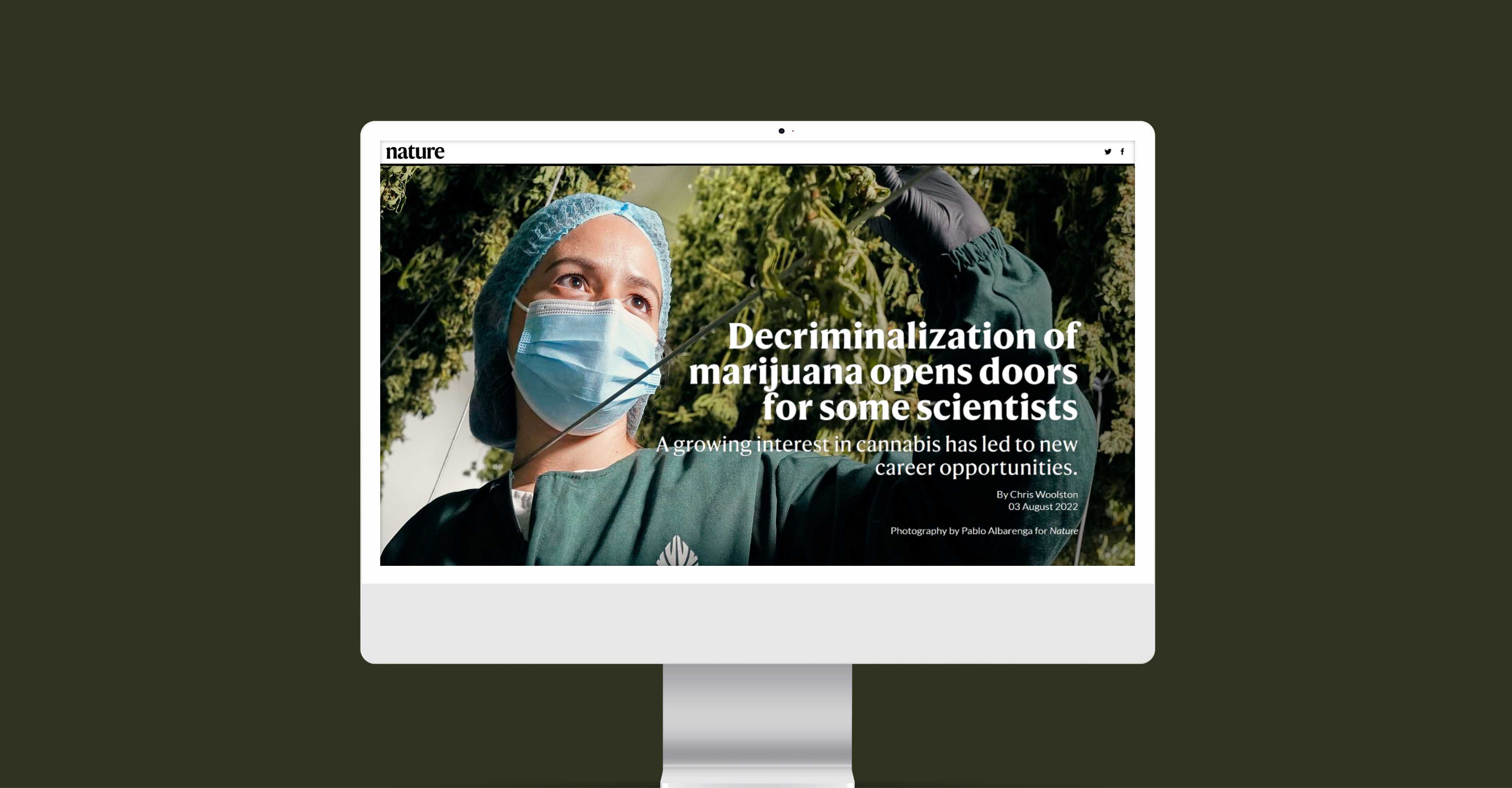The image depicts a dark gray background, with an Apple computer screen taking the forefront. Displayed on the screen is the photograph of a medical professional—a nurse—wearing light blue scrubs, a net cap or shower cap, and a face mask. She is looking upwards while stretching her gloved hand outward, seemingly inspecting something at her fingertips. The nurse is also wearing a dark green jacket. To the right of the nurse's outstretched hand, text reads, "The criminalization of marijuana opens doors for some scientists," followed by, "Proving interest in cannabis has new career opportunities." There is smaller text below the main message, providing further details. The nurse's focused gaze and the informative text capture the intersection of medical practice and evolving opportunities in the field of cannabis research.